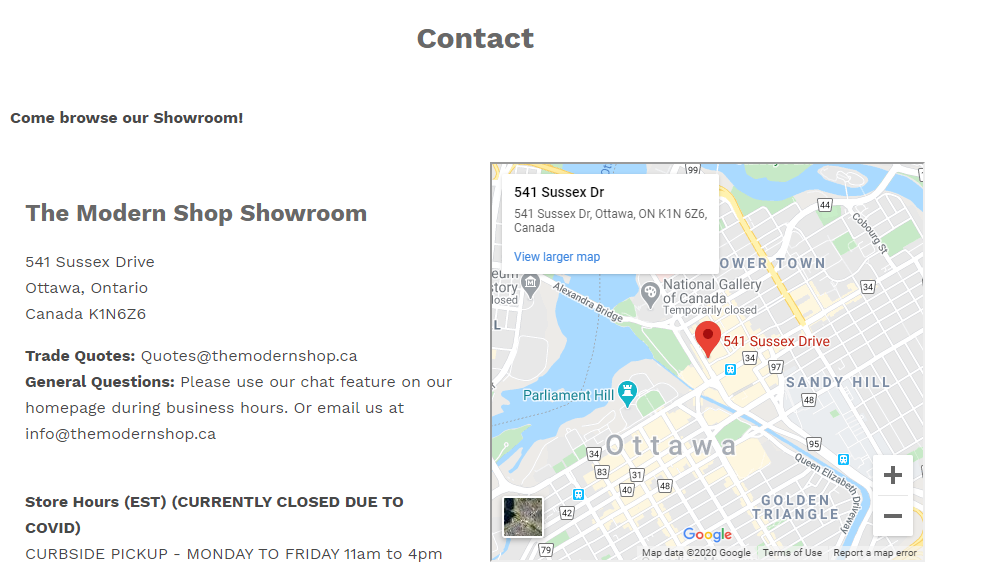On the left side of the image, a banner displays "The Modern Shoppe Showroom" with the text "Come browse our showroom" featured above it. Beneath this, in smaller text, is the address: "541 Sussex Drive, Ottawa, Ontario, Canada, K1N 6Z6." Below the address, the text continues: "For trade quotes: quotes@themodernshop.ca. For general questions, please use our chat feature on our homepage during business hours or email us at info@themodernshop.ca." Store hours are listed in Eastern Standard Time, noting that the showroom is "currently closed due to COVID-19," but "curbside pickup is available Monday to Friday, 11 a.m. to 4 p.m."

On the right side of the image, a screenshot from Google Maps is displayed, highlighting a red location pin at 451 Sussex Drive in Ottawa. The map also shows notable landmarks around the area, including Parliament Hill, the National Gallery of Canada, Sandy Hill, and the Golden Triangle.